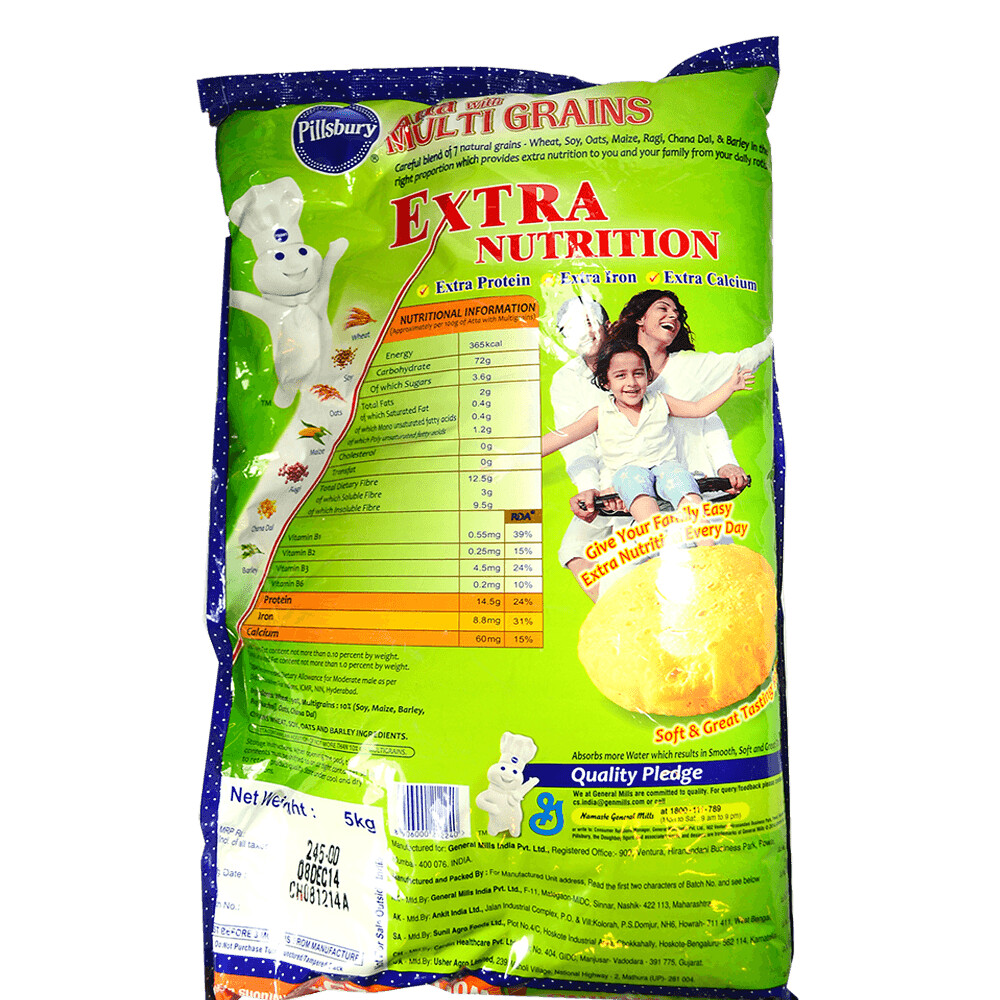The image depicts the back of a 5-kilogram package of Pillsbury Multigrains. The green and blue packaging highlights its additional nutritional benefits, such as extra protein, iron, and calcium, making it an easy way to enhance your family's daily diet. Prominently featured on the upper left-hand side is the iconic Pillsbury Doughboy, dressed in his signature white baker's hat adorned with a blue Pillsbury logo, joyfully raising his hands. The packaging also carries the Quality Pledge from Pillsbury, a member of the General Mills family, indicated by the prominent General Mills 'G' logo. This product promises not only superior nutrition but also a soft and great taste.